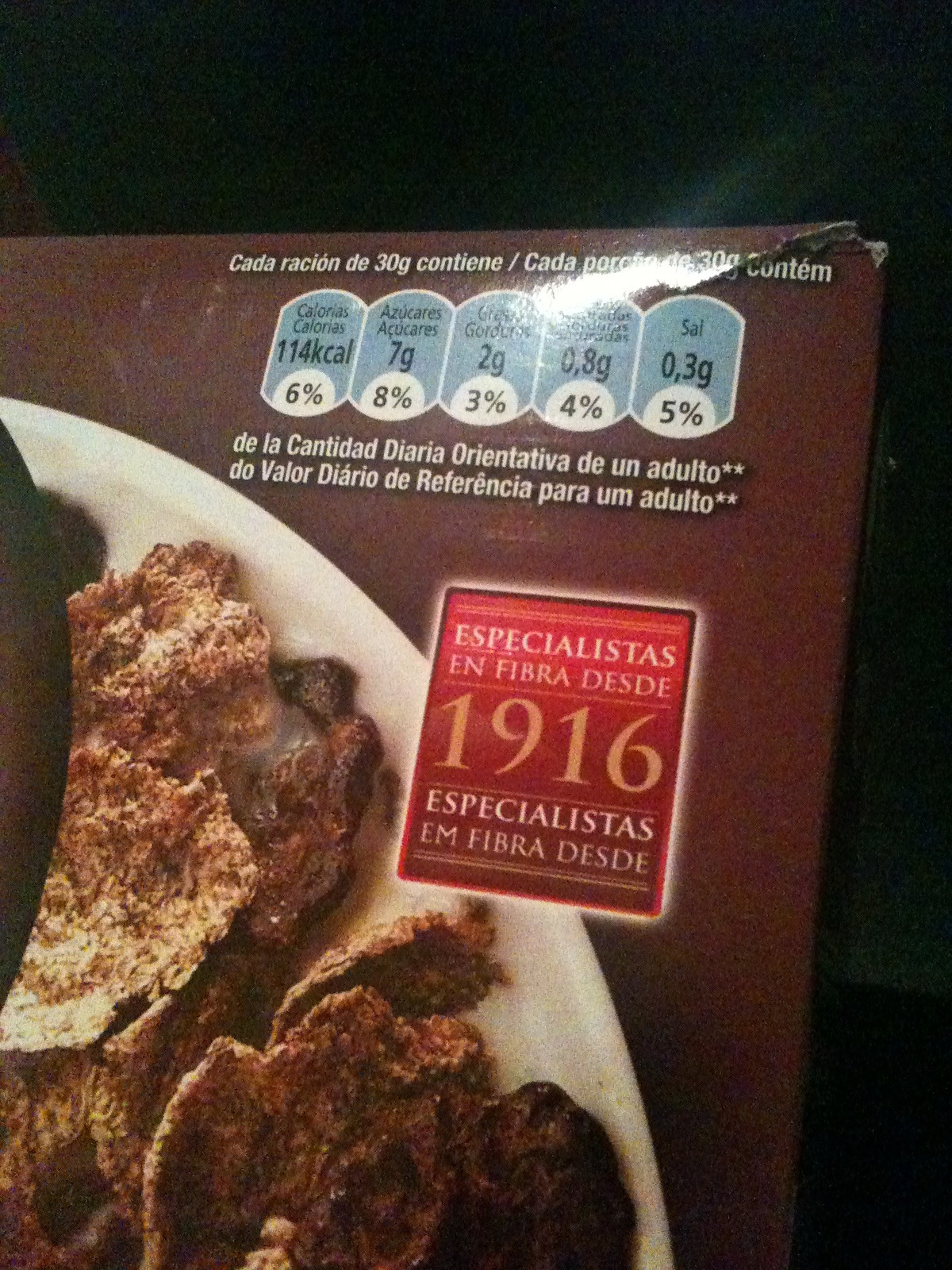This image captures the upper left-hand corner of a cardboard box, likely containing a high-fiber breakfast cereal. The box background is a deep brown, with a black backdrop. There's a white plate or bowl with dark brown flake-like objects sitting on the plate, suggesting the cereal content. Nutritional information is prominently displayed in white text on the brown background, with blue ovals highlighting values such as 114 kcal, 7 grams of "azúcares" (sugars), 2 grams of "gorduras" (fats), and 0.3 grams of salt. Unfortunately, a glare obscures part of this information, making some details illegible. A red rectangle with white and yellow text reads "Especialistas en fibra desde 1916," emphasizing the product's specialty in fiber since 1916. The text, entirely in Spanish, confirms this product is not of American origin. The top right corner of the box appears slightly torn.